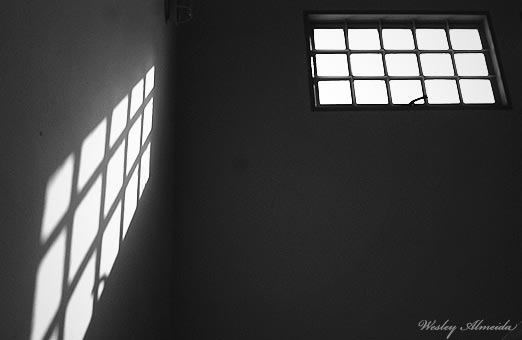This striking black and white artistic photograph captures a sunlit room, focusing on the play of light reflecting through a window. The window is situated in the top right corner of the image and features 15 glass panes arranged in three rows of five, secured with a latch at the center bottom. Sunlight filters through these panes, casting a complex pattern of light onto the opposite wall to the left. The room itself, though described as having light-colored walls, appears devoid of any actual color due to the monochromatic nature of the image. The left wall, close to the center of the photograph, also features an unlit light fixture. In the bottom right corner of the photograph, the artist's watermark "Wesley Amida" (also interpreted as "Wesley Almeida") is discreetly visible in white, semi-transparent text. The meticulous arrangement of window panes and their interaction with sunlight creates a visually appealing composition, enhanced by the grayscale palette.